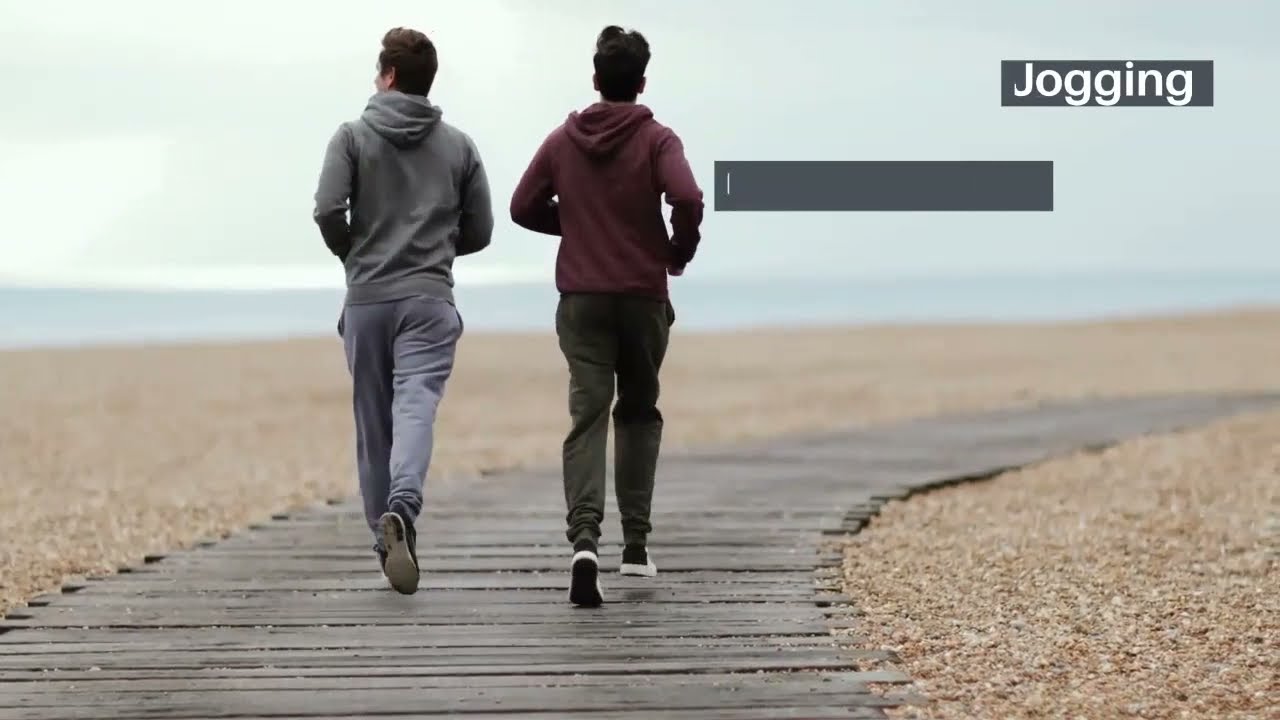A full-color, horizontally rectangular photograph captures a promotional scene set on a chilly, sandy, and rocky beach. The image, taken outdoors on a somewhat cloudy day with a slightly fuzzy background, features a light blue-gray sky and a grayish body of water in the distance. A wooden path made of long, narrow, light gray planks starts at the bottom left and curves inward toward the right, leading toward the ocean.

On this path, two dark-haired gentlemen with their backs to the camera are seen jogging. The man on the right, dressed in black shoes, black pants, and a maroon (or red) hoodie, contrasts with his jogging partner on the left, who sports black shoes, gray sweatpants, and a matching gray hoodie. Both men are immersed in their run, emphasizing the scene's dynamic nature. To the right of the image, a gray box is present with another smaller box above it, containing the word "jogging" in white letters.